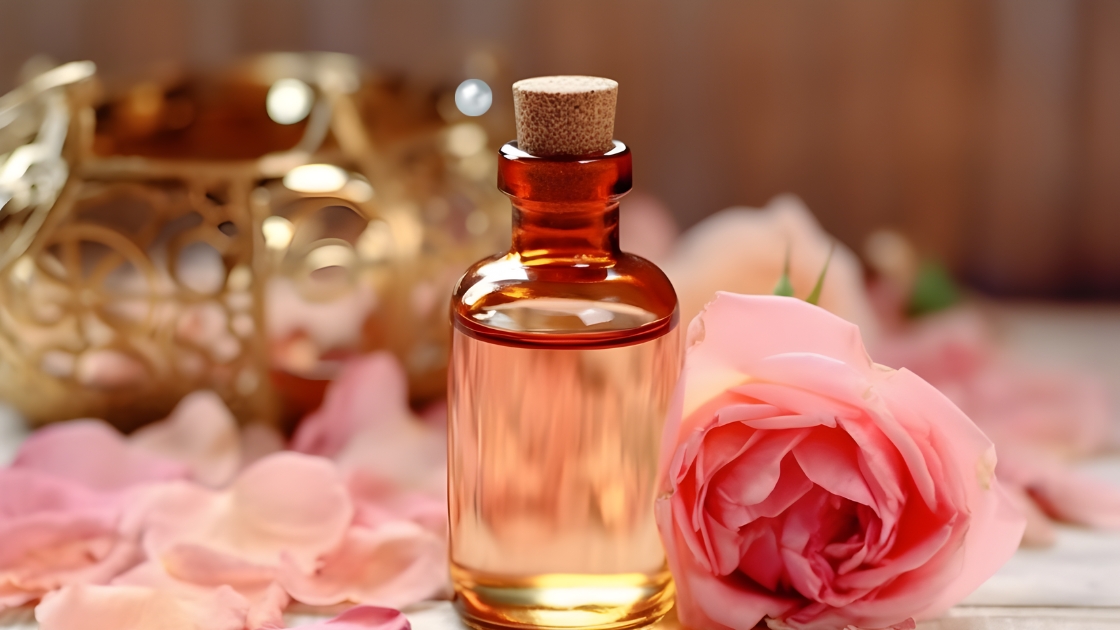The photograph captures a small, clear glass bottle with a cork stopper, which exhibits a subtle red or amber tint, particularly near its rounded top and short neck. The bottle’s wide body and thin neck are positioned centrally in the horizontal, rectangular image, extending almost from the bottom edge to near the top, revealing its clear nature as objects behind it are slightly visible. This bottle, resting on a white table or cloth, shares the scene with a full-bloomed pink rose placed to its right and scattered pink rose petals to its left. The rose and petals are in sharp focus, contrasting with the blurry background that vaguely hints at additional flowers and possibly a gold-colored decoration with circular shapes. The overall composition beautifully frames the bottle and rose, enhancing their delicate details against a softly obscured backdrop, creating an elegant and serene still-life image.